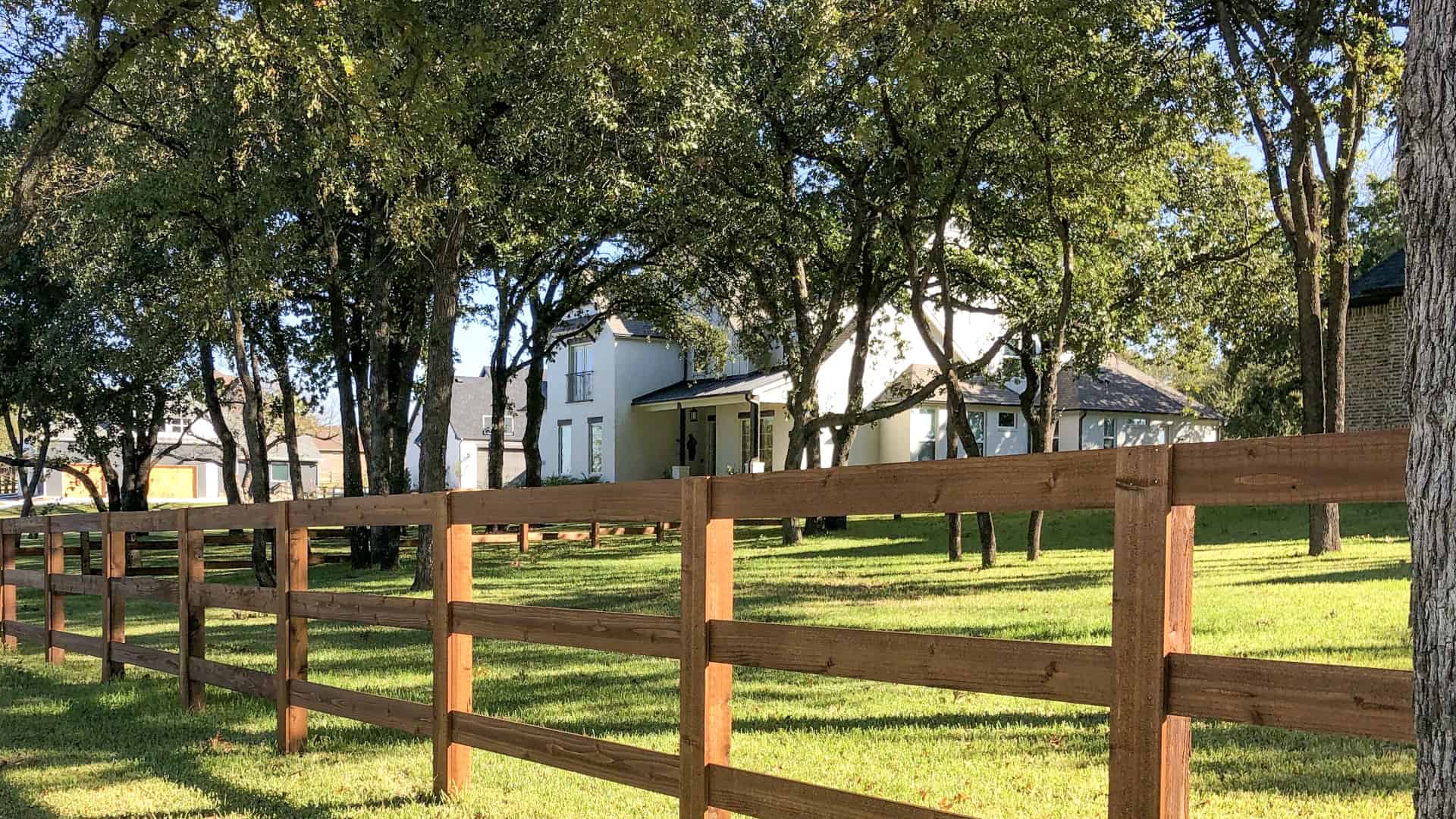This photograph captures a tranquil, sunlit scene featuring a sprawling white house with a gray roof, situated behind a line of lush green trees. The house, exuding an older, country aesthetic, highlights a small front porch and a protruding section with three windows on the right side. To the left of the porch, there are two dormer roofs with windows, adding character to the multi-story structure. In the foreground, a long brown wooden fence with three distinct horizontal slats encloses vibrant green grass, suggesting the house is fenced off for a large piece of land. To the right of the white house, a hint of a brick house peeks into view, along with glimpses of other nearby homes. The clear blue sky visible through the trees and the peaceful ambiance make the scene almost reminiscent of a farmstead, albeit without any animals present.